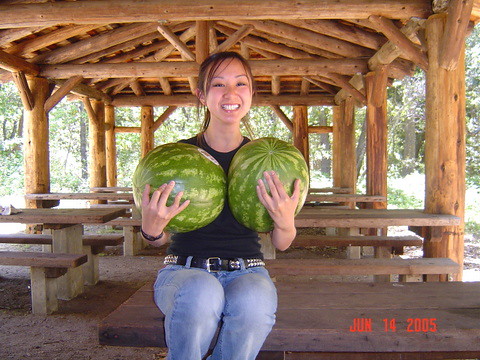In a tropical setting, a young woman sits under a robustly constructed gazebo, featuring a pitched roof supported by thick circular wooden beams and six posts—three on each side. The gazebo shelters a series of six brown picnic tables, each with benches attached to their sides. The woman, with dark hair swept to her right and pulled back, is dressed in blue jeans, a black t-shirt, and a black belt accented with metallic studs. She is smiling broadly, holding two massive watermelons in front of her chest with her hands positioned at the front. A black watch adorns her right wrist. Surrounding the gazebo is a fully filled-in tree line, devoid of any buildings or other people, enhancing the secluded, natural atmosphere.